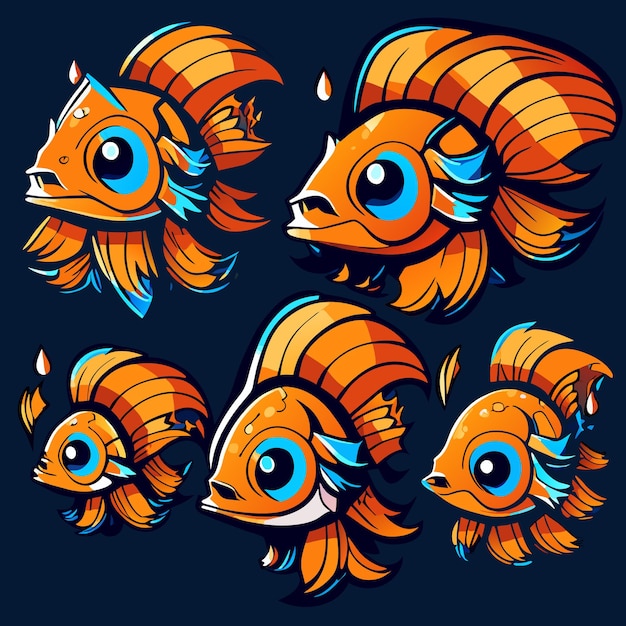This stylized illustration depicts five goldfish, all oriented to the left against a deep blue backdrop. The fish differ slightly in size, with two larger ones on top and three smaller ones below, evoking a parent-child dynamic. Each goldfish, rendered in varying shades of orange—from bright and light to almost brownish—features prominent, flowing fins and blue accents, including striking blue eyes. The fish are drawn in a consistent, vector-like style, appearing almost identical at first glance, with subtle distinctions. The scene also includes a few floating elements resembling water droplets, adorned with white and orange highlights. The overall effect resembles a pop art wallpaper, evoking a playful and vibrant aquatic scene.